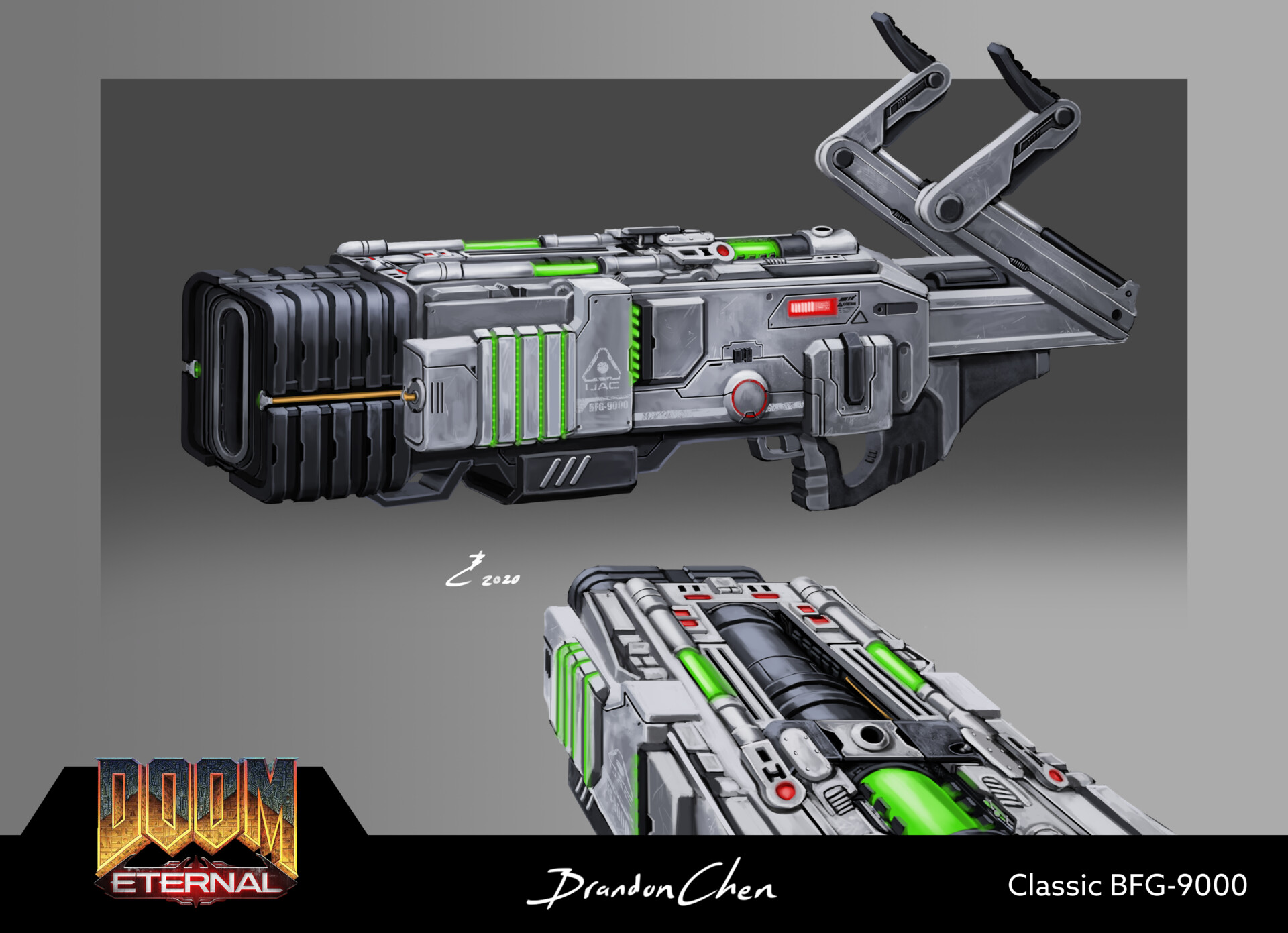The image is a detailed advertisement for the video game "Doom Eternal" featuring a hand-sketched depiction of the iconic weapon, the Classic BFG 9000. The prominent "DOOM" lettering is emblazoned with a fiery orange, yellow, and red gradient. Below this, the word "Eternal" is outlined in a reddish hue. The weapon itself is a massive, futuristic design built in 2020, featuring a square silver metal body with lime green accents and additional mechanical gadgets. It has a small trigger at the bottom, suggesting a unique and cumbersome hold, possibly requiring two hands or shoulder mounting. The image shows two versions of the weapon: one is centrally sketched with meticulous detail, indicating a heavy and complex build, while another is pointed away towards the dark grey background. The entire scene is annotated with "Doom Eternal" on the bottom left, artist "Brandon Chen" in the center, and the label "Classic BFG 9000" on the bottom right—all dated 2020 with a white signature.